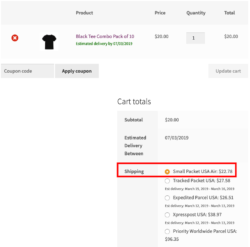The image is a screenshot of an online shopping cart displaying a black short-sleeved T-shirt, identified as "Black Tee Combo Pack of 10." The interface shows detailed information and actions related to the shopping cart. At the top, there's a red "Save" button partially covering some text that reads "Product" across the header. Following this, columns are labeled "Price," "Quantity," and "Total." Below this, there is an "X" icon allowing for item deletion. The price is blurred but appears to be between $30 and $36, with a quantity listed as one.

To the left, beneath these details, are boxes for entering a coupon code and an adjacent "Apply Coupon" button. Further to the right is an "Update Cart" button. The cart totals section shows a subtotal, which is likely around $26, and an estimated delivery date that includes the year 2019. Shipping options are displayed, with the selected method highlighted in a red box, although the shipping cost remains unclear. Additional shipping options are listed below the selected one.